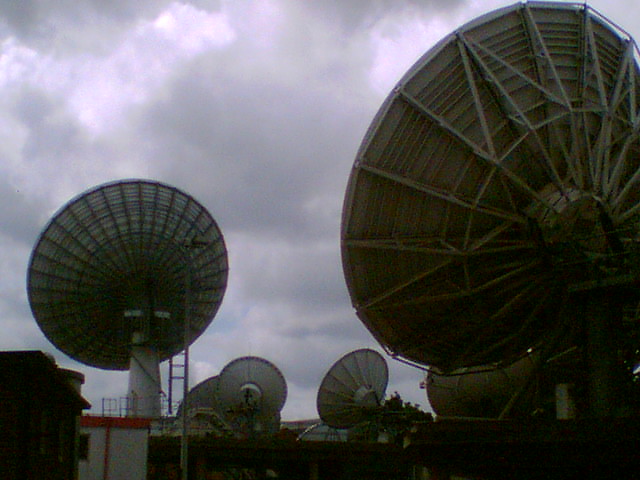This image captures a cluster of satellite dishes of varying sizes, all positioned towards an overcast sky. Dominating the right side of the frame, a gigantic satellite dish features concentric circles and is supported by triangular structures. On the left, further away, another prominent dish with radiating spokes and an attached ladder is visible. Scattered between these two large dishes, there are smaller dishes in the background, summing up to about five or six in total. The scene also includes a white building with red trim and a red roof, visible beneath the satellite dishes. In the lower left-hand corner, the obscure silhouette of another building emerges, details obscured by shadow. Vegetation silhouettes along the horizon. The sky above is heavily overcast with no blue sky visible, casting a muted light over the entire scene.